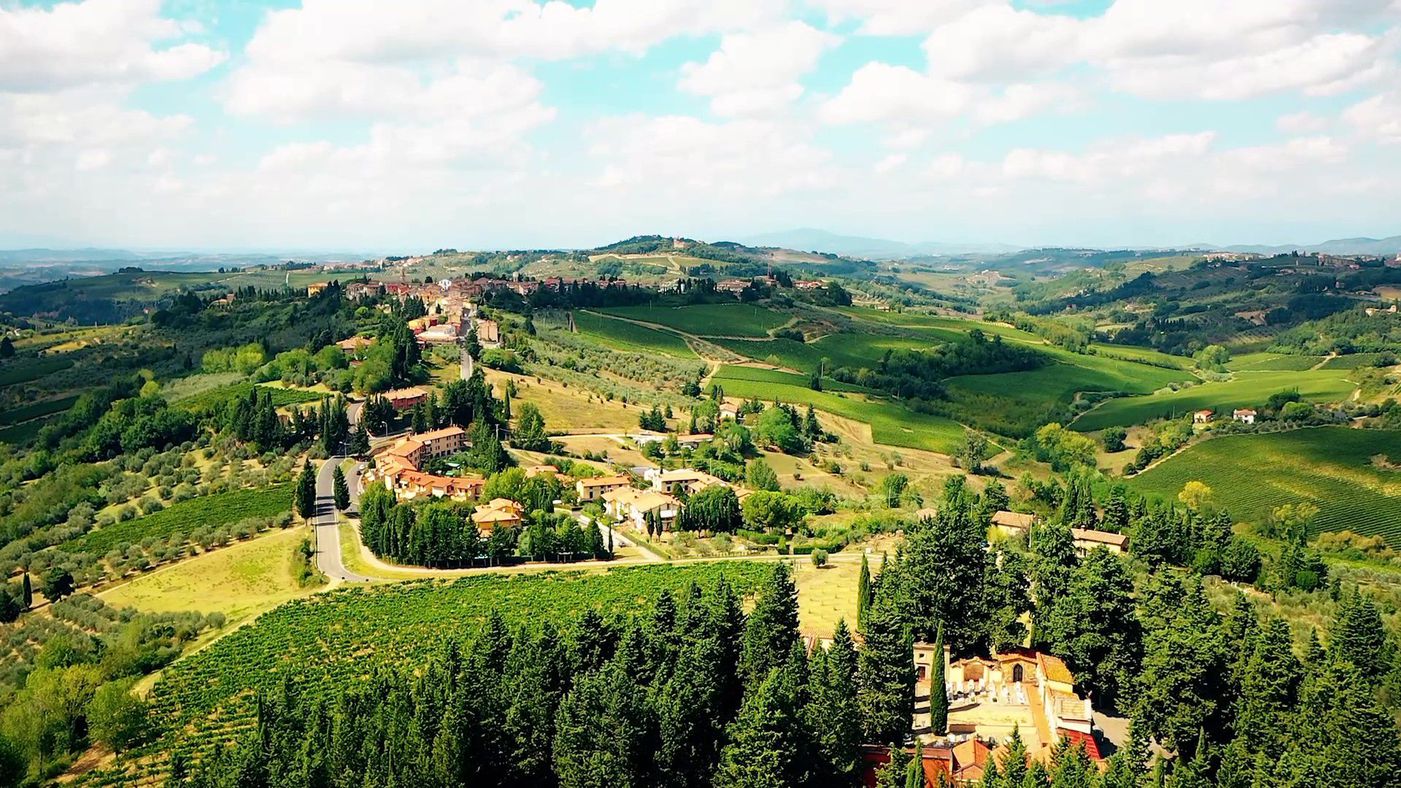This aerial photograph vividly captures a lush green countryside characterized by rolling hills and elevated terrains. The landscape features a mix of dense evergreen trees and expansive grassy areas interspersed with weeds. Dominating the center-left, there is a noteworthy circular building surrounded by trees and encircled by distinct yellow pavement. This area is connected via a steep descending road to another cluster of red brick buildings with white roofs, which are also framed by evergreen trees. The entire scene is set against a picturesque backdrop of a blue sky filled with numerous puffy white clouds, highlighting the vastness and tranquility of this historic and seemingly remote hillside locale.